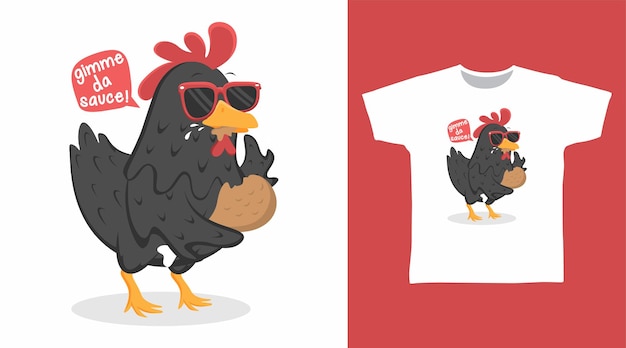The image is a clip art-style illustration divided into two panels. The left side of the panel features a black chicken with red sunglasses, gleefully eating a fried chicken leg in a cannibalistic manner. A speech bubble emanates from the chicken's beak, stating "Gimme Da Sauce," suggesting a desire for possibly spicy sauce, as a drop of sweat near its beak indicates discomfort. The chicken has red highlights on its head and a distinctive red wattle. The right side of the panel displays a white T-shirt with the exact same chicken graphic printed on it, set against a vivid red background. This suggests that the design is available for purchase on a T-shirt, likely intended as fun merchandise, possibly for a chicken-themed restaurant. The overall quirky and creative artwork, featuring the cool-looking, sunglasses-wearing chicken, makes it an attractive and humorous product.